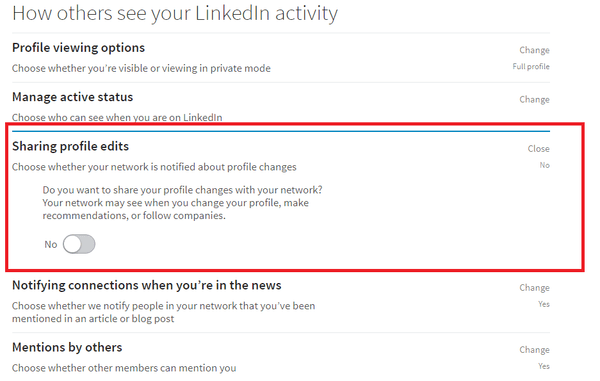This detailed image captures a section of either a LinkedIn mobile app or website. The background is entirely white. In the top left corner, "How Others See Your LinkedIn Activity" is displayed in a slender gray font. Below this, there's a small gap before the title "Profile Viewing Options" appears prominently in bold black font. To the far right of this title, in a smaller gray font, the word "Change" is visible.

Beneath "Profile Viewing Options," a subtext in gray font reads, "Choose Whether You Are Visible or Viewing in Private Mode." Lower down on the bottom left-hand side, "Manage Active Status" is written in bold black font. Directly below, in gray font, the text says, "Choose Who Can See You When You're on LinkedIn." On the far right-hand side, once again, the word "Change" is present.

There is a red, thin, yet noticeable rectangular box encompassing the section titled "Sharing Profile Edits" in bold black text. Inside this section, the text in gray slender font reads, "Choose Whether Your Network Is Notified About Profile Changes." Underneath, there is a toggle button with the question, "Do You Want to Share Your Profile Changes With Your Network?" The accompanying description notes, "Your network may see when you change your profile, make recommendations, or follow companies." A circular button offers a toggle option between "no" and "yes."

Below this section, in bold black font, the heading "Notify Connections When You're in the News" appears, followed by a gray-font description, "Choose Whether You Will Notify People in Your Network That You've Been Mentioned in an Article or Blog Post." The final heading, "Mentions by Others," is in bold black font, and its accompanying gray text states, "Choose Whether Other Members Can Mention You."